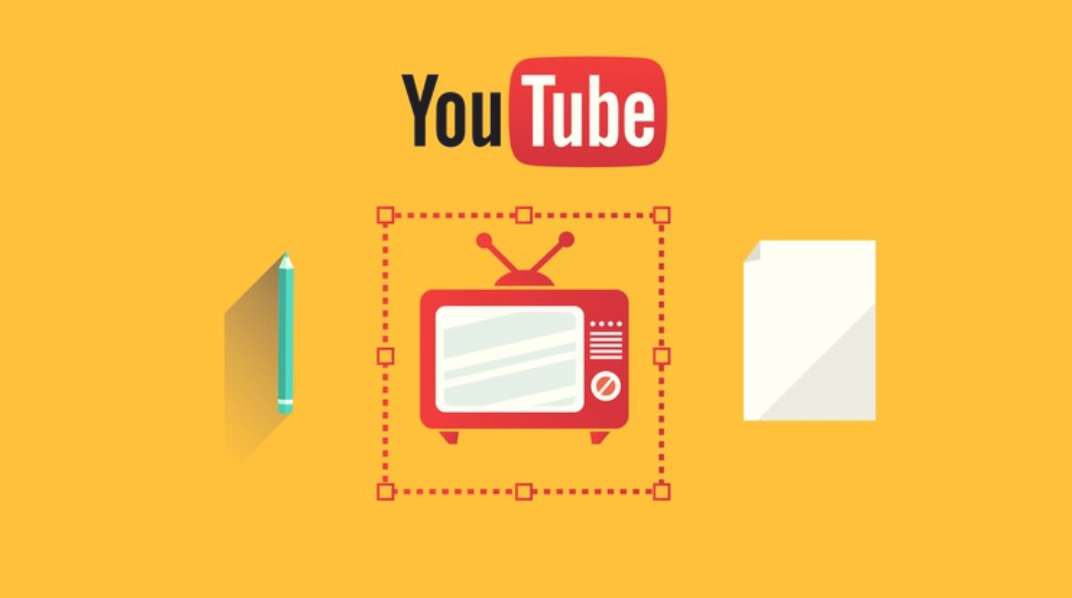The image features an advertisement for the YouTube brand set against a plain yellow background reminiscent of mac and cheese. Central to the image, three objects are prominently displayed. On the left side, there is a blue pencil. In the middle, an old-style TV with antennas and knobs stands out, enclosed within a dotted-line box, suggestive of a selection tool in graphic design software. To the right, a blank sheet of paper is shown. The iconic YouTube logo, with the word "You" in black text and "Tube" in white encased within a red rounded rectangle, is positioned at the top of the image. The detailed selection box around the TV, complete with squares at the corners and center, indicates that the TV is the focal point, as if it were selected for adjustment in a digital interface.